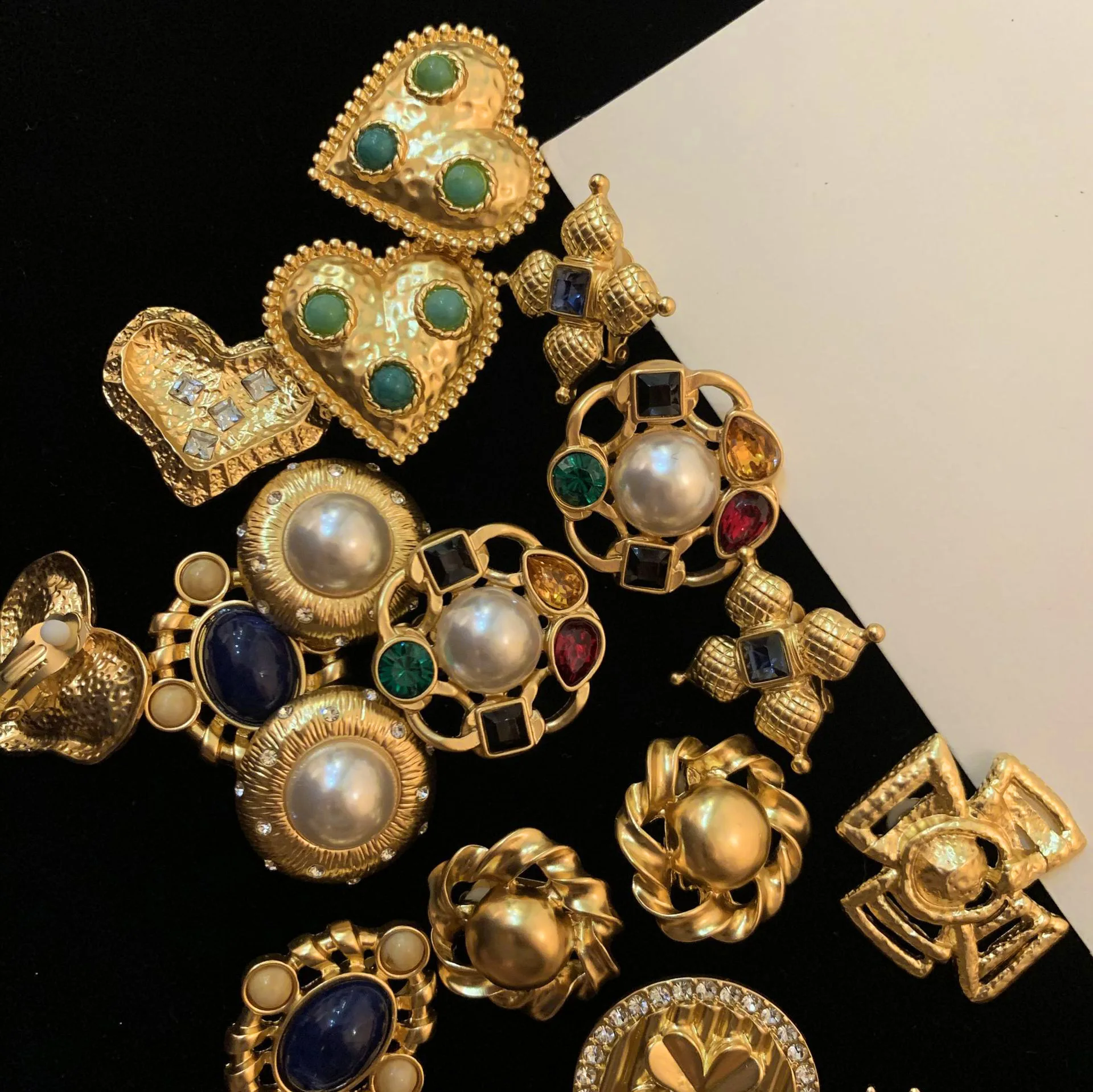The photograph displays an assortment of ornate golden jewelry, likely brooches or pins, carefully arranged on a black surface. Among the collection are several heart-shaped pieces adorned with vibrant green gemstones, and two circular brooches with a central pearl surrounded by a variety of gems, including orange, red, black, and green stones. A standout piece features a large central pearl encircled by an intricate pattern. There's also a piece with a dark navy blue oval gem, adding a touch of deep elegance to the assortment. Another notable item is cross-shaped with a square gem in the middle. This curated selection of about 12 to 15 pieces rests alongside a piece of white paper extending from the upper right-hand corner to nearly the lower right-hand corner of the image. The detailed embellishments and diverse shapes suggest a rich display of artistry and craftsmanship.